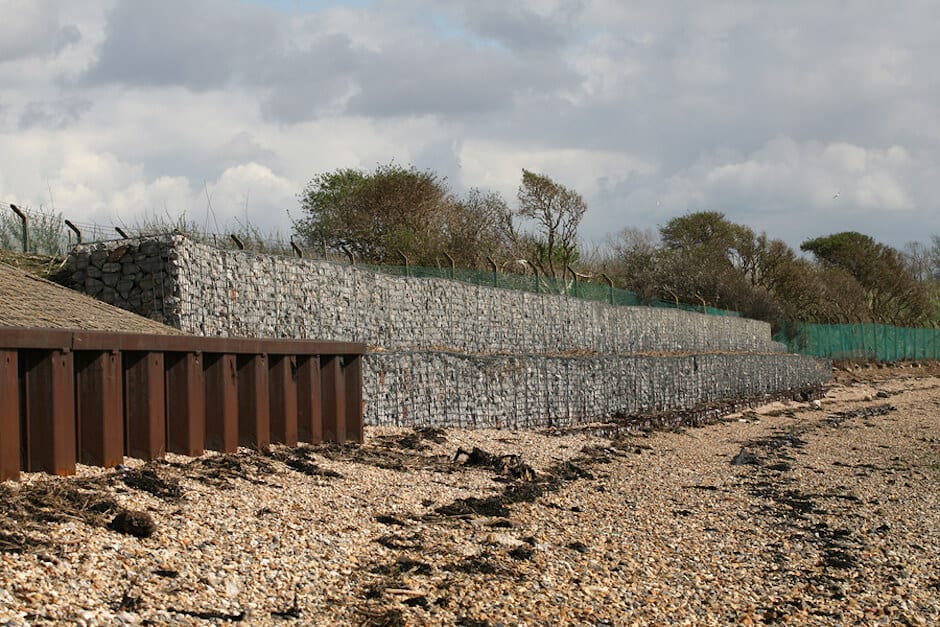The photograph depicts a rugged, rocky shoreline, possibly a stone beach, with various forms of debris such as plants, seaweed, and perhaps shells scattered across tan and beige stones. The sky is mostly cloudy with occasional blue patches, casting a bright yet overcast ambiance. Dominating the midsection of the image is a tiered structure that resembles a dam or retaining wall. The left side of this structure features rusty steel planks, while the middle portion consists of metal cages filled with rocks, lending to the image's industrial feel. Adjacent to these structures is a severe-looking green security fence topped with barbed wire. Bordering the horizon, several trees stand tall, adding a natural contrast to the otherwise man-made scene.